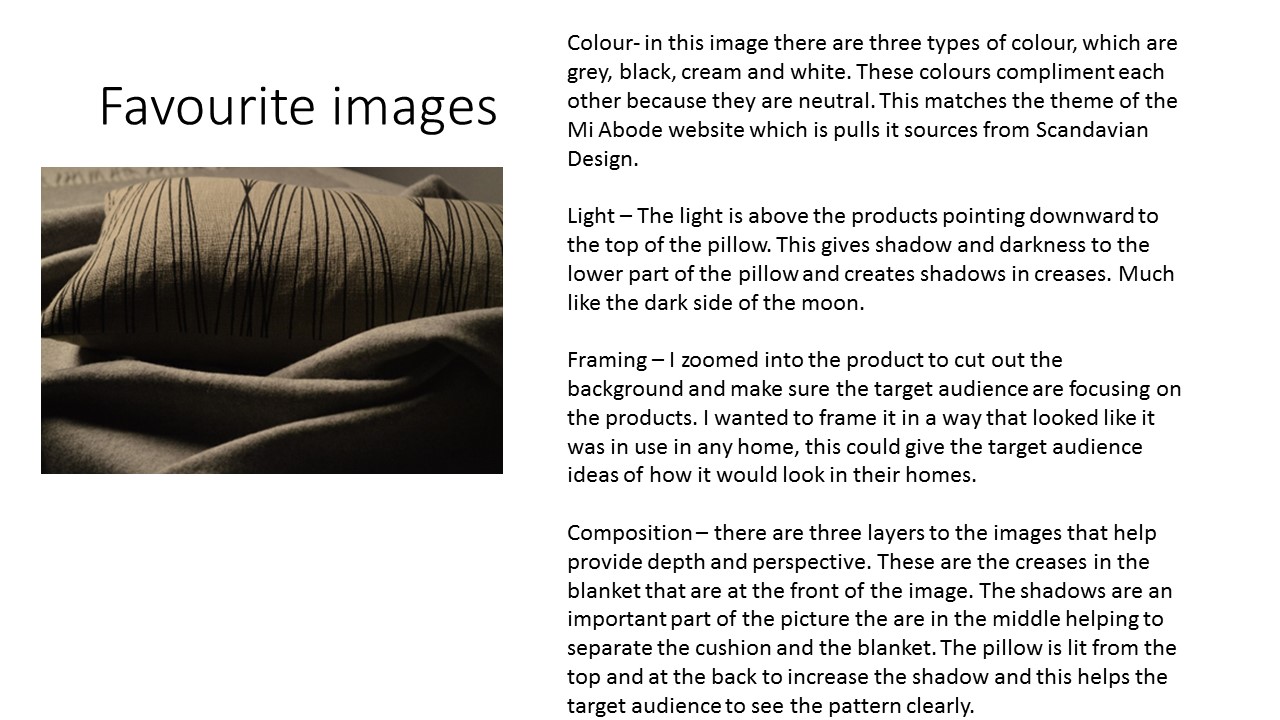The image depicts a pillow adorned with black stripes on a tan background, resting atop a folded sheet, both in varying shades of tan. Above the photograph, the text "Favorite Images" is prominently displayed in black. The image background is white, enhancing the visual clarity. The accompanying text description is positioned to the right of the photograph, structured into four sections: Color, Light, Framing, and Composition, all printed in black. The color section discusses the use of gray, black, cream, and white, highlighting how these neutral tones complement each other and draw inspiration from Scandinavian design. The light section elucidates that the pillow is illuminated from above and behind, creating shadows that accentuate the pattern. The detailed text emphasizes the careful consideration of lighting, framing, and composition, suggesting that the image could be suitable for display in a museum or as an instructional piece.